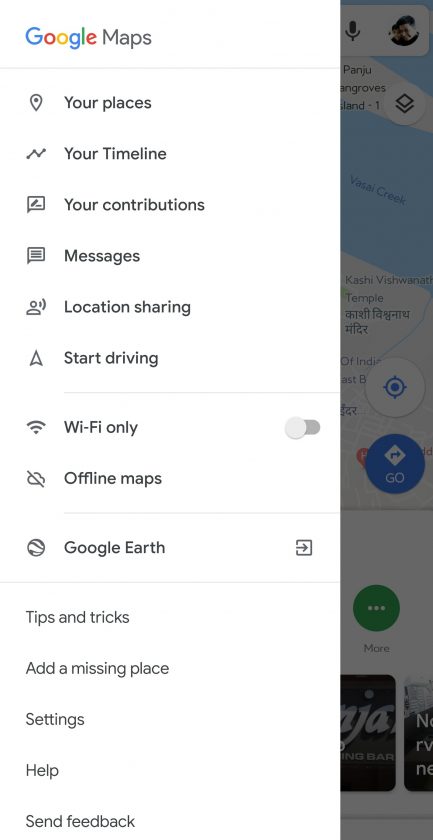This image depicts the user interface of the Google Maps application. At the top, the iconic Google logo is displayed in its vibrant colors—blue, red, yellow, and green—followed by the word "Maps" in black font. Below the logo, a variety of categories are listed, each accompanied by its own icon. These categories include: "Your places," "Your timeline," "Your contributions," "Messages," "Location sharing," "Start driving," "Wi-Fi only," "Offline maps," and "Google Earth," with the last three featuring additional interactive elements like switches and arrows pointing right.

Towards the bottom section, additional options such as "Tips and Tricks," "Add a missing place," "Settings," "Help," and "Send feedback" are available. On the right-hand side of the webpage, there is a narrow, greyed-over map strip. The map is not clear and appears darkened, making it difficult to discern details without closer inspection. 

At the top of the map, a microphone icon is visible, indicating voice search capabilities. The map itself shows some water bodies and a central blue circle labeled "Go," representing a starting point or a location pin. Additionally, there is a green circular icon with three white dots, labeled "More," suggesting more options or settings. 

At the bottom of the interface, there are two partially visible cards, likely advertisements, but they are cut off, making their content indiscernible.